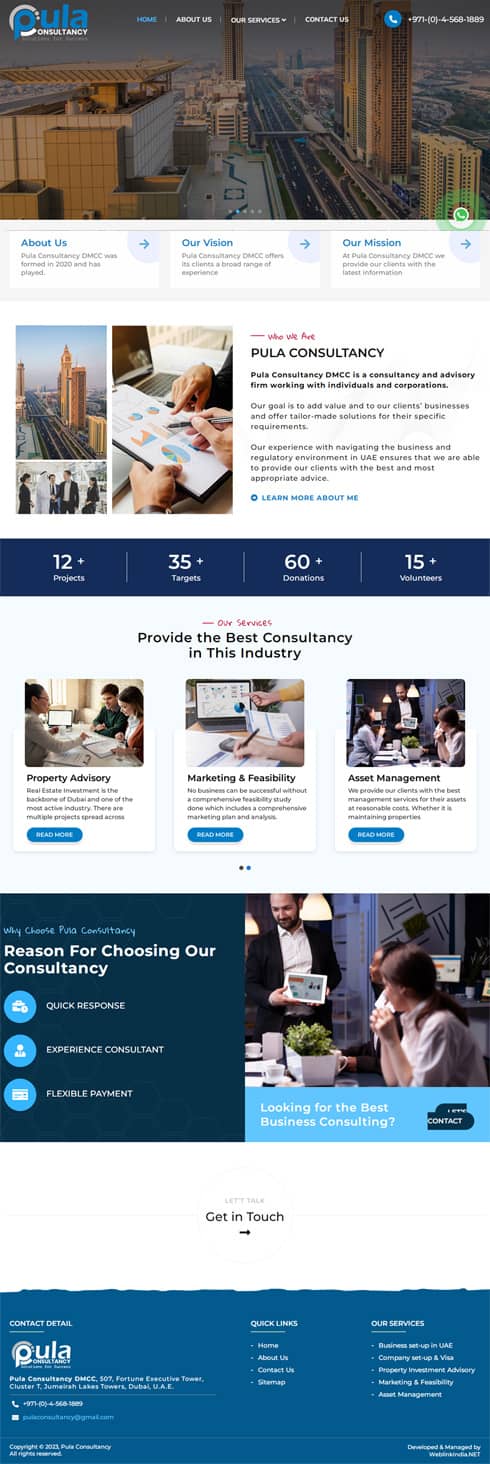The image depicts a detailed webpage layout for the "Pula Consultancy" website, which is designed in a way that resembles an iPad screen.

### Header:
- **Cityscape Background**: The top 20% of the page features a cityscape with skyscrapers and buildings. 
- **Title and Sub-title**: At the center, it says "Pula Consultancy" in blue, with a smaller font below it spelling "consultancy."
- **Navigation Options**: Various menu options are aligned across the top.
- **Contact Information**: In the far right corner, there is a blue circle with a phone icon and a phone number, though the font is too small to read clearly.

### Main Content:
- **Three Primary Boxes**:
  - **About Us**: Contains information about the consultancy.
  - **Our Vision**: Details the company's vision.
  - **Our Mission**: Outlines the company's mission.

- **Who We Are Section**:
  - Includes a picture of cityscape and people discussing issues.
  - Showcases a man holding an iPad with graphs on it.

- **Pula Consultancy Description**:
  - To the right, it has a detailed text block about Pula Consultancy.
  - Below the text, there are four blue rectangles with white text stating: 
    - "12+ Projects"
    - "35+ Clients"
    - "60+ Donations"
    - "15+ Volunteers"
  - The text in these boxes is somewhat small and hard to read.

### Services Section:
- **Three Boxes on White Backgrounds**:
  - **Property Advisory** (People talking at a table)
  - **Marketing and Feasibility** (Man looking at graphs and writing something)
  - **Asset Management** (People talking at a table)

### Reasons for Choosing Pula Consultancy:
- Blue box listing:
  - "Quick Experience"
  - "Quick Reference"
  - "Experienced Consultancy"
  - "Flexible Employment"

- Adjacent Picture:
  - Man holding an iPad showing graphs.
  - People sipping coffee and discussing around a table.

### Footer:
- **Get in Touch Section**: 
  - Blue box stating contact details for Pula Consultancy.
  - Three columns:
    - **Quick Links**: Includes four bullet points.
    - **Our Services**: Includes five bullet points.

This comprehensive layout is both detailed and organized, showcasing the various aspects and offerings of Pula Consultancy clearly, although some text elements are noted as small and difficult to read.